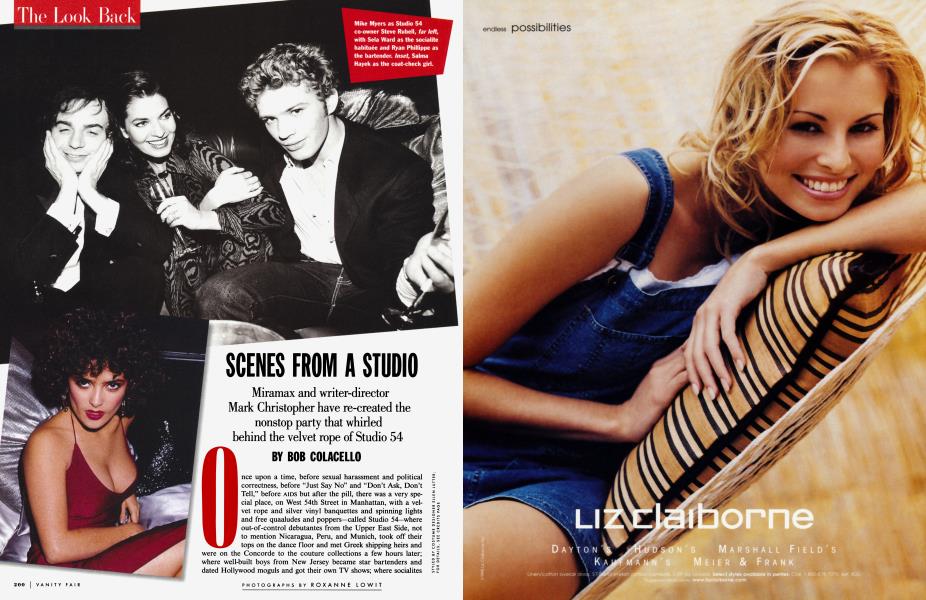This is an open spread from Vanity Fair magazine, featuring an article on the left page and a Liz Claiborne advertisement on the right. The advertisement on the right showcases a smiling, blonde-haired, tanned Caucasian woman leaning against a cushioned chair. Her hair is parted in the middle and styled in a crinkly, wavy manner. She wears a blue tank top suit that reveals her brown skin, and her hands rest on the cushion of the chair. The text "Liz Claiborne" is written in white letters near her chin. 

On the left page, there is an article titled "Scenes from a Studio" by Bob Colacello, highlighted by a black and white image of three people: Mike Myers, a woman with her hands crossed, and another man with curly hair, likely Ryan Phillipe. At the bottom left corner of the left page, there's a color photograph of Salma Hayek in character, with black curly hair and a low-cut amber dress showing significant cleavage. Her hands are positioned in front of her stomach. The top corners of the article contain red sections with white text, though the text is too small to discern. A large red letter "O" starts one of the paragraphs, and "Vanity Fair" with an unreadable page number is visible in the bottom left corner.